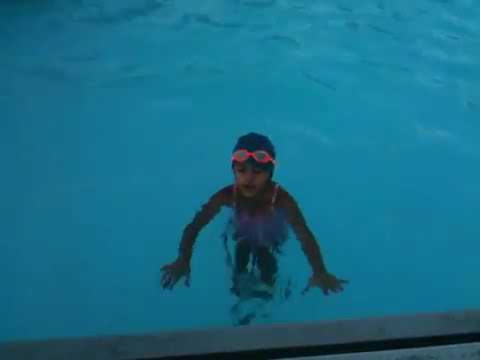In this photograph, we see a young girl with light brown skin in a swimming pool, captured from above. The pool's vivid blue water fills nearly the entire frame, with only a hint of the light gray pool edge visible at the very bottom. The image quality is quite low, with noticeable visual artifacts. The girl, positioned toward the bottom center of the square image, appears to be wading with her arms outstretched under the water. Only her head and shoulders emerge above the surface. She wears a dark swim cap with bright pink goggles resting just above her eyes. Although her swimsuit is partially obscured and blurry underwater, it seems to be pink as well. The overall scene emphasizes the blue water and the girl's distinct swimwear, framed in a simple, clear pool setting.